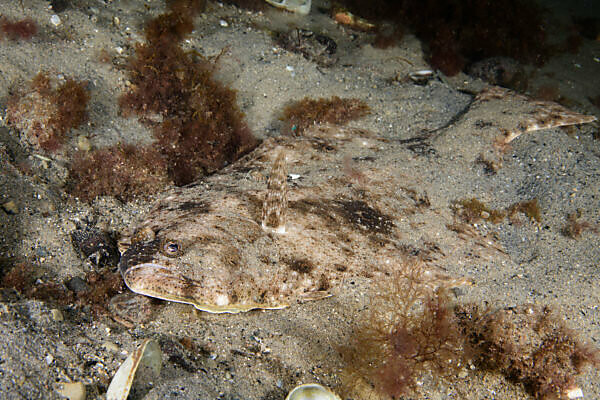This underwater photograph, despite being low-resolution and heavily compressed, captures a sandy seafloor or lake bed with various plant life. The central focus is a flat, elongated fish, likely a type of flounder, partially buried and camouflaged within the sand. The fish's sandy coloration, speckled with brown and black, blends seamlessly with the mixed tan, gray, and brown sand particles, as well as the surrounding moss and algae. Notably, the fish exhibits a visible eye and mouth in the middle of the image, with a fin adorned with frilly, brownish filaments on its top left side. A faint white line around its neck area distinguishes the head from the body. The image appears to have been taken in the dim depths of the sea or lake, illuminated by a light source to reveal the fish against the darker top-right background. The fish's body stretches diagonally across the picture, occupying about a third of the frame.